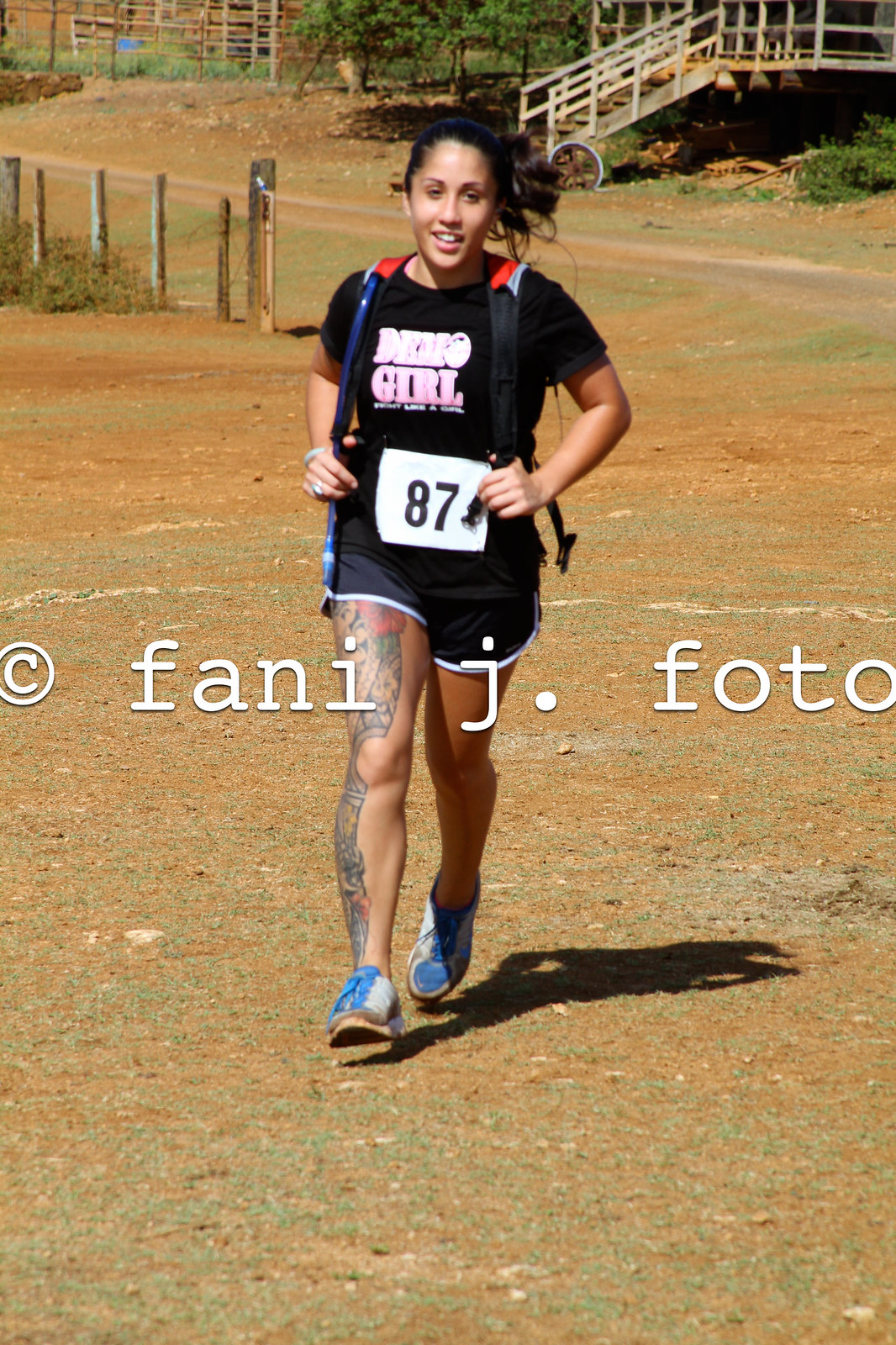This outdoor photograph captures a young woman, possibly in her late teens to early twenties, running on a dirt road, likely competing in a race or marathon. The ground she's running on is predominantly tan pebbles and pale brown material, with sparse grass and small bushes visible. She has long black hair tied back in a ponytail and is dressed in a black short-sleeved t-shirt with "Demo Girl" written in pink letters on the chest. A white square with the number 87 is pinned to her belly. She wears black shorts with white trim and blue and white running shoes. The setting includes some trees, a pale wooden fence to the upper left, and a staircase with a wooden railing leading up to a deck on the upper right. The woman has a long tattoo running from her thigh to her ankle. She is front and center in the photo, smiling as she runs. A watermark in the center of the image displays "© Fani J. Foto."